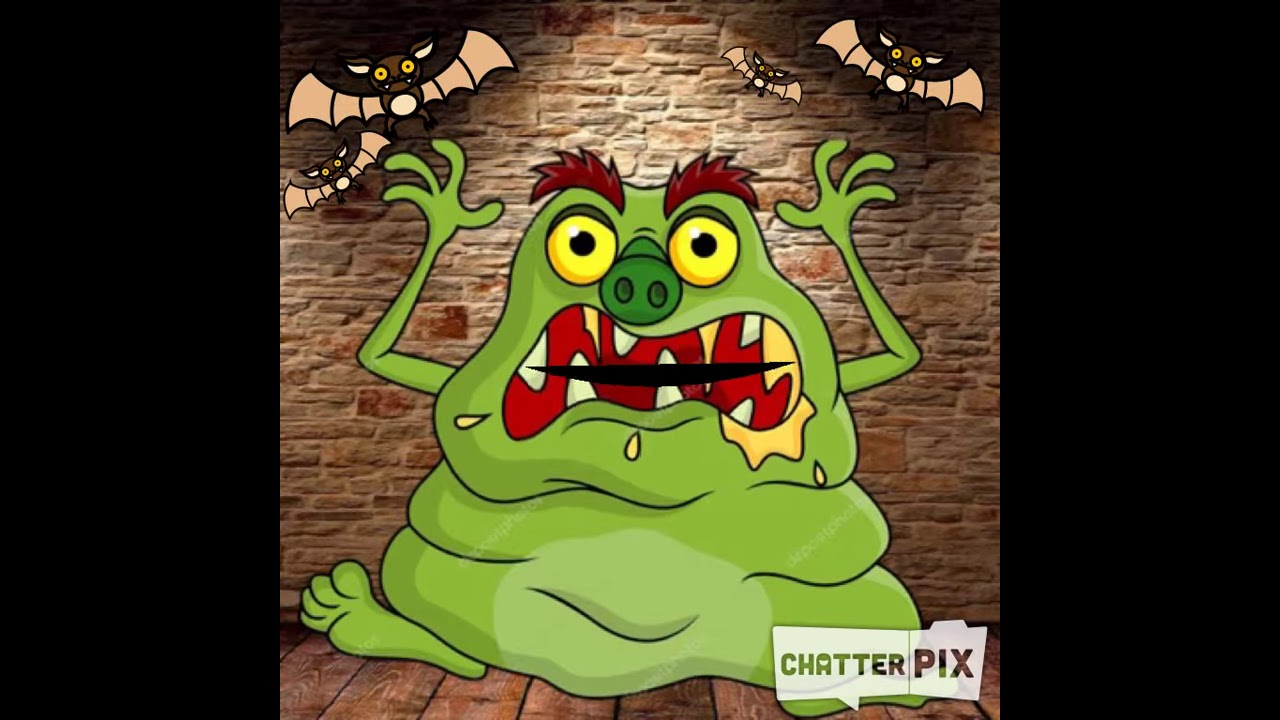This is a detailed, animated cartoon image featuring a comically grotesque green blob monster with prominent yellow eyes and a pig-like snout. The monster displays a mouthful of spaced-out, crooked teeth with slobber visibly hanging from the sides. Sporting furry brown eyebrows and raising his slimy green hands in a wide, exaggerated gesture of surprise or fear, his overall appearance is more humorous than frightening. The monster stands on a wooden floor against a backdrop of a brown brick wall. In the top part of the image, four animated bats with beige wings, brown bodies, and bright yellow eyes hover menacingly. Notably, in the bottom right corner, there's a white rectangle with the word "ChatterPix" inscribed, marking the possible source of the animation. The setting and characters suggest a whimsical take on a spooky, Halloween-esque theme, with the goofy-looking blob monster at its center.